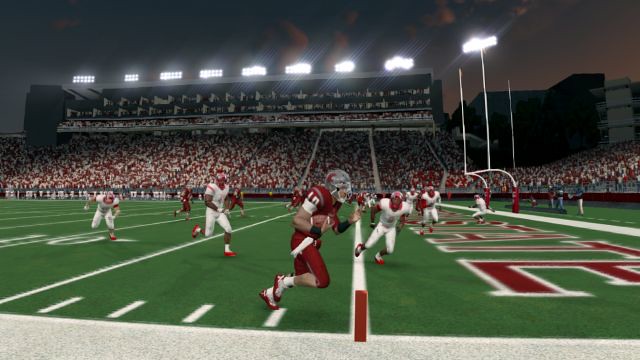The image depicts a football game set in a stadium brimming with spectators. At the focal point near the goal line, a player donned in a red jersey, red pants, and matching gear is seen charging towards the end zone, firmly clutching the football as he aims for a touchdown. Peculiarities within the image hint at its artificial origins, either from a low-resolution video game or AI generation.

Notably, a bank of field lights is improbably mounted atop the goal post in the upper right corner, an impossible anomaly in real-world stadium setups. The faces of the opposing football players in white uniforms appear unnaturally distorted, missing essential facial features. Similarly, the audience in the grandstands, although numerous, has an eerily uniform appearance, displaying a salt-and-pepper look indicative of a repetitive pattern. This repetition is particularly evident in the center of the grandstand, where a distinct pattern of a hook-shaped white figure followed by a triple white shape recurs.

Additional irregularities include smeared writing in the end zone, where the lines are not straight and the letters have blurred edges, further corroborating the likelihood of AI construction.